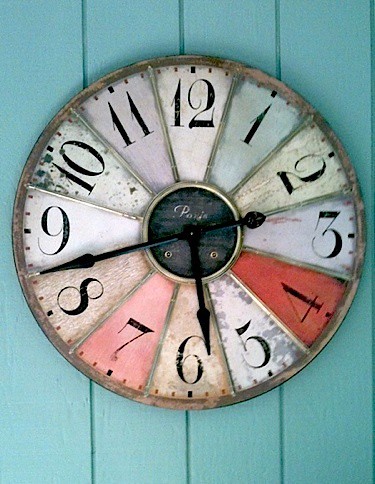This image features a rustic round clock with a weathered, possibly wood frame, mounted on a robin's egg blue wood-paneled wall, which is divided into four vertical sections by three thin lines. The clock's face is split into twelve pie-shaped sections, each uniquely colored in muted tones like tan, white, a fair blue, light green, red, pink, and purple. These segments correspond to the numbers 1 through 12, which are displayed in black font. The black metal hour and minute hands, pointed at the ends, indicate the time is 5:43. At the center of the clock face, there is white text that appears to say "Paris." The clock, though colorful, carries an aged and slightly dirty appearance, reflecting its rustic charm.